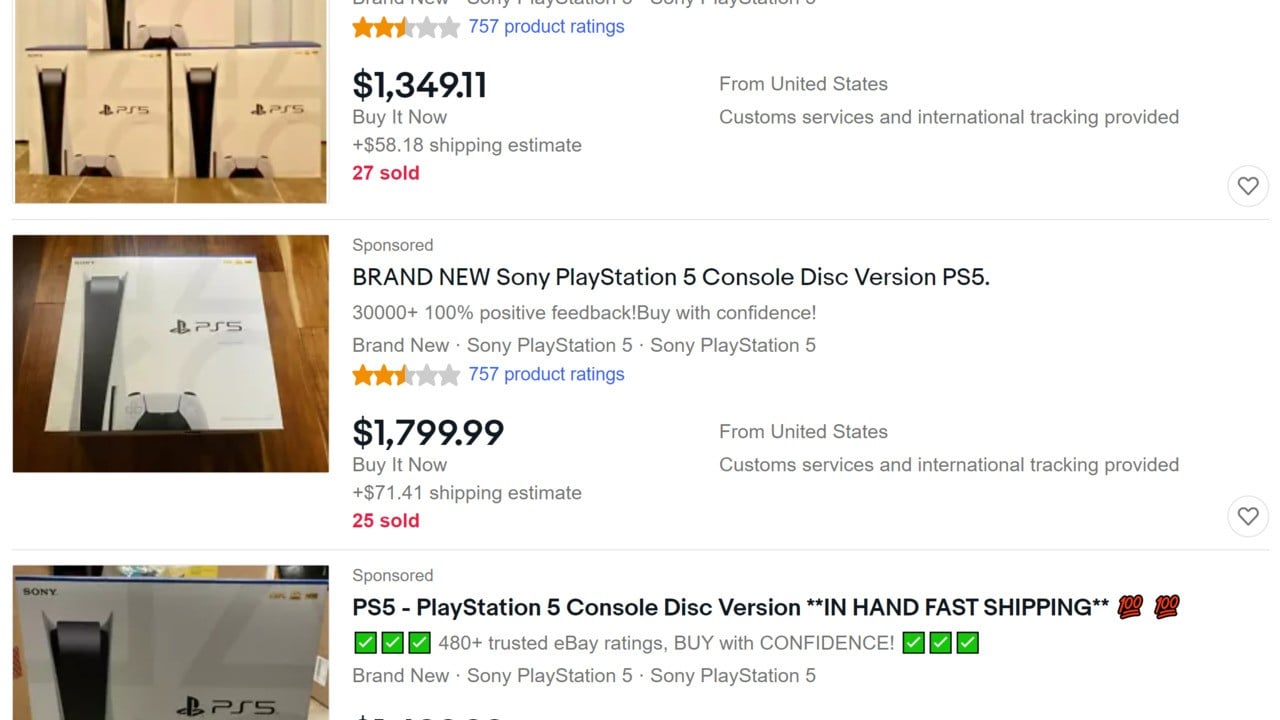A screenshot of a website, possibly eBay, features listings for PS5s being sold through a bidding system. On the left side, images of the PS5 consoles are displayed, while on the right, their prices are listed. The top listing shows a price of $1,349.11, the middle listing is priced at $1,799.99, and the price of the bottom listing is cut off and unviewable. Each listing includes shipping estimates, with all three originating from the United States, though details for the bottom listing are partially cut off. The listings offer a "Buy It Now" option. Reviews show both the top and middle listings having a 2.5-star rating based on 757 product ratings each. The top listing features multiple PS5 boxes in its image, whereas the middle and bottom listings each show a single PS5 box. A green checkmark box is visible on the bottom listing, indicating a form of approval or verification.